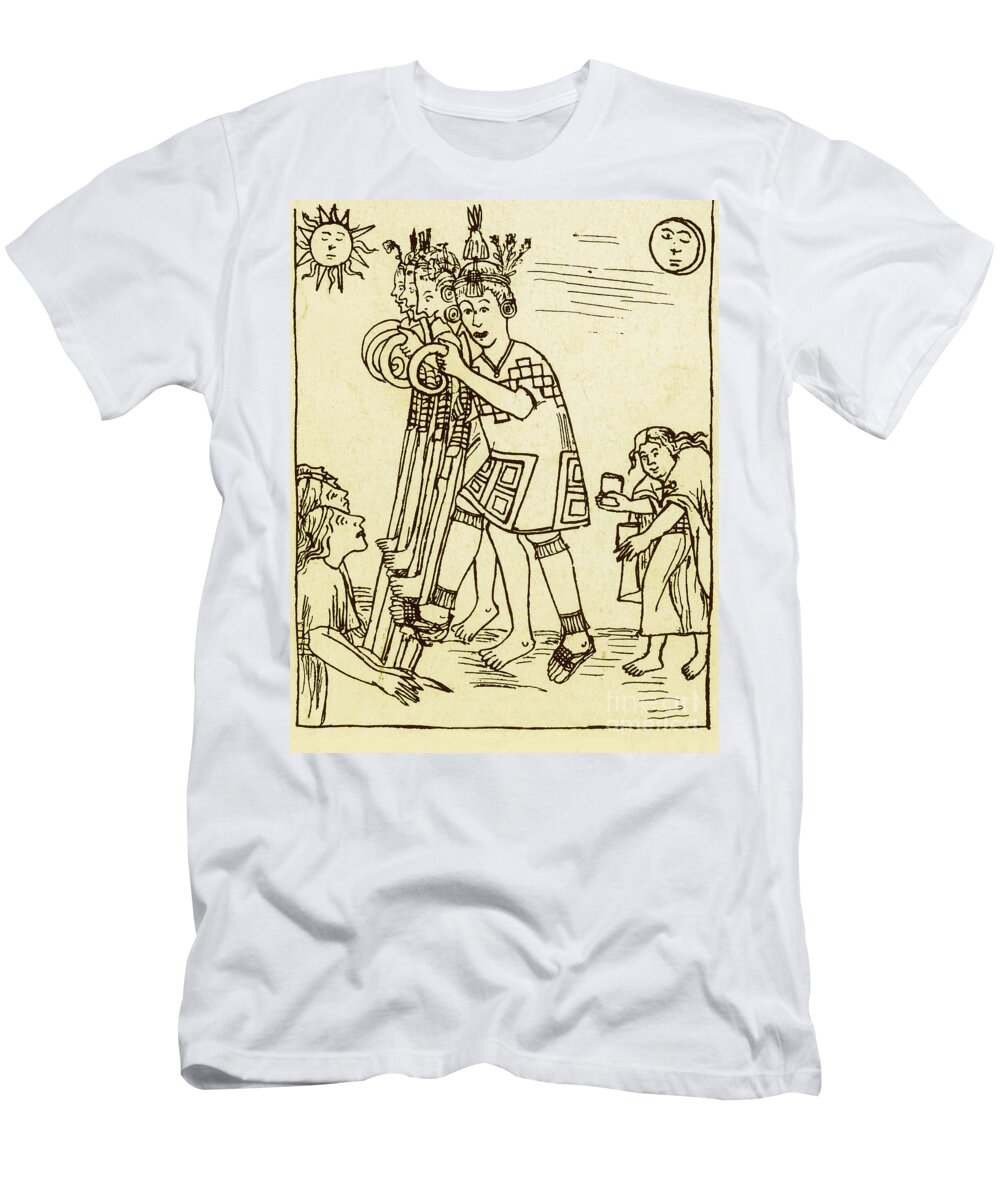This image depicts a wrinkled men's short sleeve crewneck t-shirt, without a visible neckline tag. The t-shirt is a light tan color and features a vertical rectangle graphic on the front, resembling aged parchment. This graphic is primarily black line art and showcases a scene with sketched figures that appear to be ancient or indigenous people. The background of this artwork includes a sun in the top left corner and a moon in the top right, both with faces. 

In the center of the graphic, various female characters are walking in a straight line. Some of them are barefoot, while others wear sandals, and they are adorned in headdresses and outfits with geometric patterns. Their bodies blend together, making it difficult to distinguish each individual character. On the right side of the scene, a lady appears to be hunched over as if rushing towards the group, while on the left side, two women observe the procession. The figures in the center, possibly children, seem to partake in some form of competition, suggesting a possible race or contest involving sticks or stilts with curved handles. This intricate representation adds a rich, narrative quality to the otherwise simple garment.